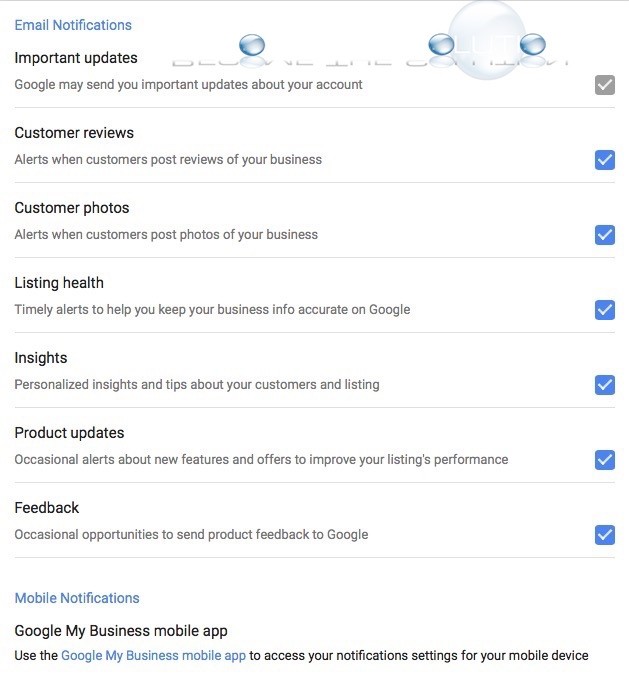This image appears to be a screenshot from a website, likely pertaining to Google My Business notification settings. The background is predominantly white, and a thin light gray line stretches across the top of the page, lending subtle structure to the layout.

At the top, the header features "Email Notifications" in blue text. Directly beneath this, in bold black font, is the sub-heading "Important Updates," followed by a brief description: "Google may send you important updates about your account." 

To the right of this section, there are a series of blue speech bubbles accompanied by white check marks inside gray boxes, all separated by gray divider lines. These icons likely indicate selectable options.

Following the "Important Updates" section, the next category is "Customer Reviews," succeeded by "Customer Photos," with an explanation: "Alerts when customers post photos of your business." Next, there's "Listing Health," which provides "Alerts to help you keep your business info accurate on Google."

Below this category, the next section is labeled "Insights," described as "Personalized insights and tips about your customers and listing." Further down, another category exists for "Product Updates," and lastly, "Feedback."

Each category has a blue box on the right side with a white check mark, indicating default or user-selected options.

At the bottom of the image, the "Mobile Notifications" section is introduced, specifying "Google My Business Mobile App." The description provided states: "Use the Google My Business mobile app to access your notification settings for your mobile device."

The meticulous structure and segmented layout of this page likely aim to facilitate easy navigation and clarity for users managing their Google My Business notification preferences.